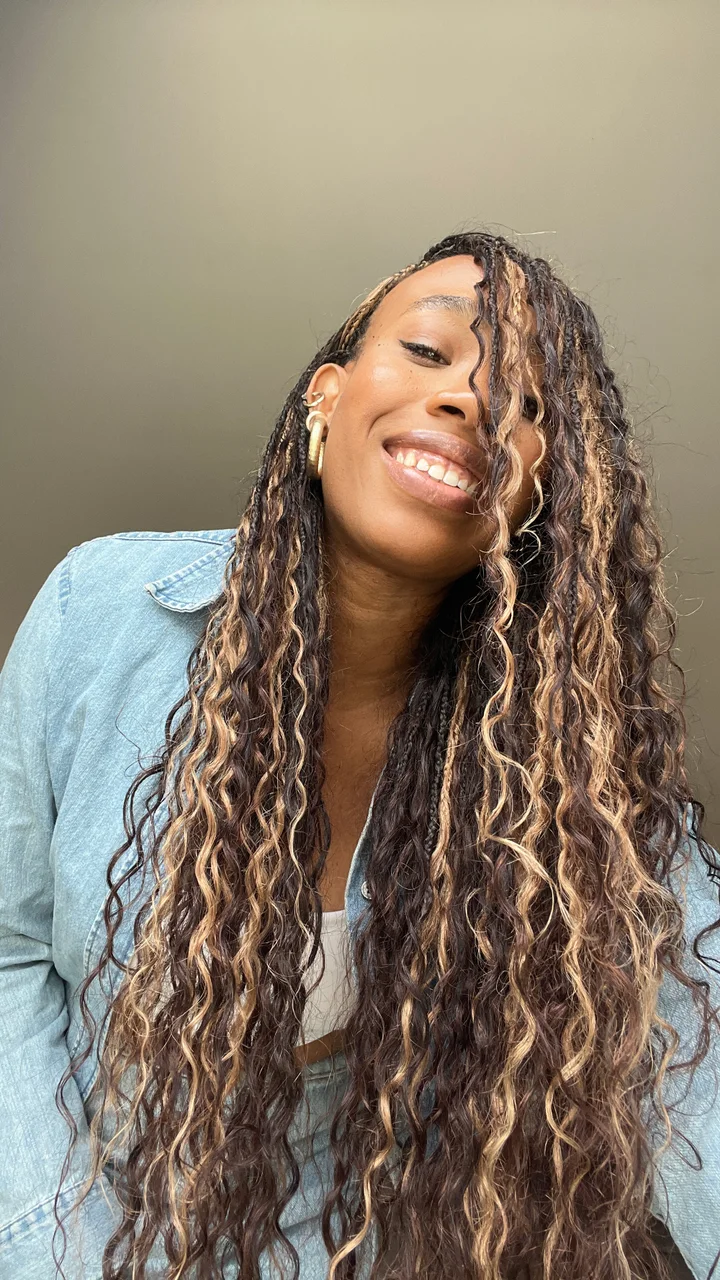The photograph captures a beautiful African American woman with medium-light skin tone, smiling warmly as she looks slightly down into the camera, suggesting a selfie. She is adorned with natural makeup, displaying a touch of lip gloss and eyeliner, which enhances her radiant and happy appearance. Her exceptionally long, wavy, and curly dark brown hair, interspersed with lighter blonde highlights, cascades past her waist, extending beyond the frame of the image. She is dressed in light wash denim from head to toe, featuring a button-up shirt or jacket, and either pants or a skirt, paired with a white bandeau top. The simplicity of the background, a plain gray wall, ensures that all attention remains on her. She accessorizes with an array of gold earrings, including a large hoop in each ear and smaller ones higher up on her earlobes. The photograph is taken from a lower angle, adding to the engaging composition of the image.